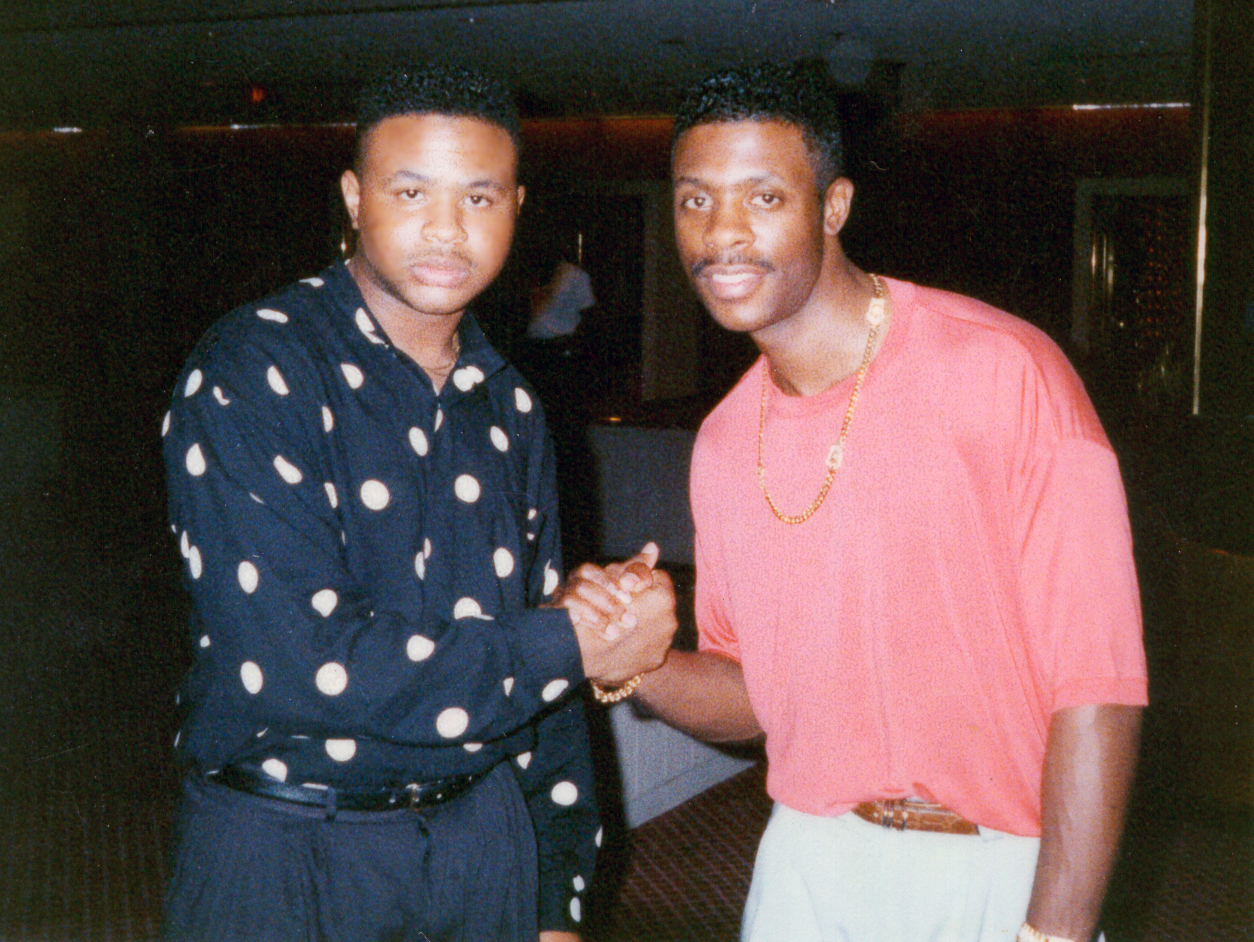In this 1980s-style photograph, two black men are shaking hands and facing the camera in what appears to be a dimly lit indoor venue, possibly a strip club. The man on the right is dressed in a tucked-in salmon-colored shirt paired with white pants and a brown leather belt. He accessorizes with gold bracelets on each wrist and a gold chain necklace, and sports a pencil mustache. The man on the left wears a long-sleeved, black shirt adorned with white polka dots, tucked into black pants held by a black belt. The dark background features a gold pole on the right side, contributing to the gritty, vintage aesthetic captured by a strong flash. The varied color palette includes shades of coral pink, beige, khaki, dark blue, white, black, maroon red, and gold. Both men are looking directly at the camera, with vague silhouettes suggesting other individuals in the distant background, emphasizing the intimate yet enigmatic atmosphere of the scene.